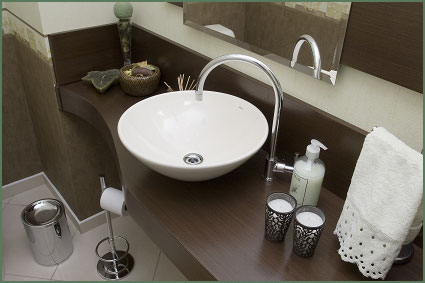This image showcases a pristine and organized bathroom sink area, possibly within a hotel. The floor features white tiles, contributing to the clean and bright ambiance. A small, silver tin trash can, reminiscent of those often found in hotels, is strategically placed. Resting on the floor is a toilet paper holder made of silver metal, comprising a circular base, a supporting pole, and another ring to hold the roll.

The upper half of the wall is painted white, while the lower half is brown, adorned with white trim. The counter is constructed from dark chestnut wood, starting narrow and then extending outward in a curvy, bottle cap-like design where the sink is located. On the left side of the counter, a decorative frame hangs above a leaf-shaped tray and a large ornamental pot.

The sink itself is bowl-shaped, with a clear view of the drain and a long, curved faucet. Reflected in a small mirror above the sink, details such as a white soap dispenser and two candles resting in brown, intricately designed cups are visible. Additionally, a white towel with fringes and decorative holes is elegantly hung on a holder similar to the toilet paper stand, likely intended for face or hand washing. This well-appointed and aesthetically pleasing bathroom space embodies both functionality and style.